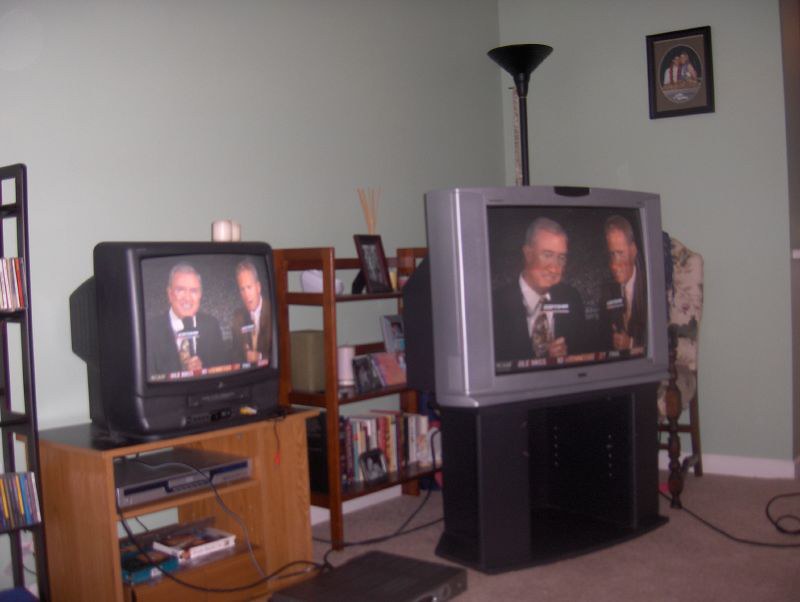The image is a color photograph from the early 2000s, capturing a corner of a living room with a muted green wall adorned with white baseboard trim. The prominent feature is two CRT televisions, both tuned to the same station displaying two older men with gray hair and microphones, likely sportscasters, with a slight millisecond delay on the right TV. The smaller, black TV on the left sits on an oak wood entertainment center with two shelves housing a VCR and various VHS tapes. Adjacent to it is a larger, silver TV on a dark gray or black stand. Between the two TVs, a DVD player is on the floor, connecting to both devices with visible cables. The room also includes a black torchiere lamp in the corner, wall-to-wall carpeting, and a picture of two people hugging, or potentially a framed record album, on the wall. Additional elements include a CD rack on the far left, a low bookcase of likely teak wood with books, photos, and vases on its three shelves, adding a nostalgic charm to the scene.